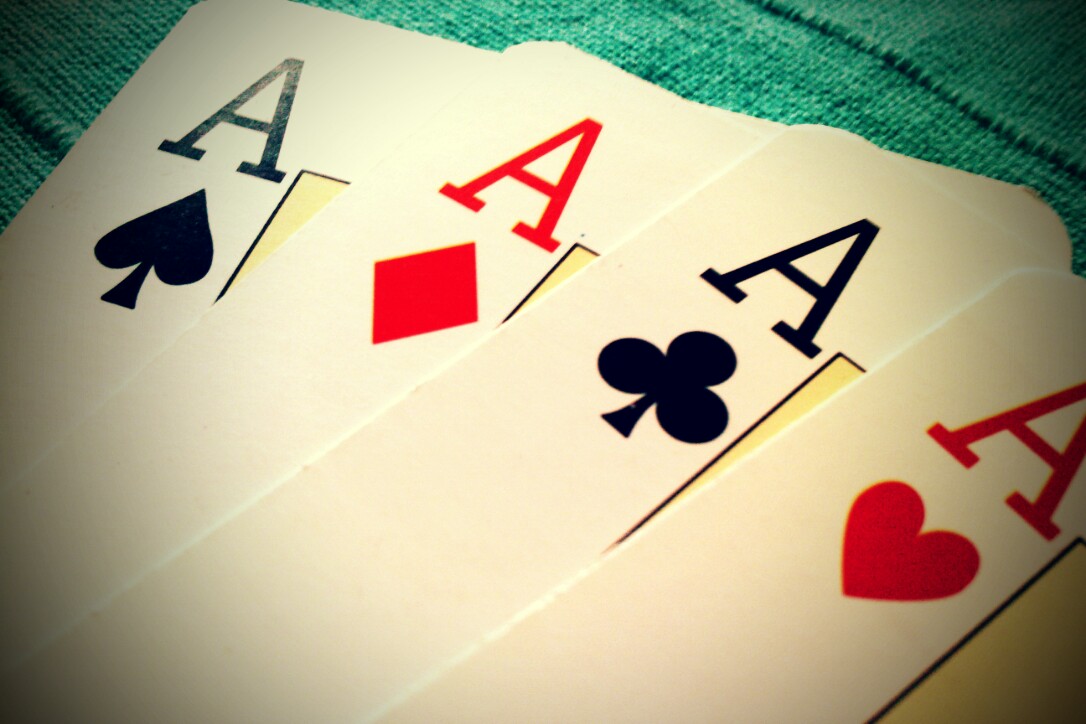A close-up photograph showcases a quartet of overlapping aces from a deck of playing cards, arranged meticulously on a solid green, textured fabric that features subtle ridges. The ace of spades sits predominantly on the left side, its upper-left corner extending to the top of the image, leaving no green fabric visible in that spot. Decorated with a black "A" and spade symbol, it is partially covered by the ace of diamonds, which displays a red "A" and diamond emblem. Further overlapping in the sequence is the ace of clubs, featuring a black "A" and club symbol, positioned from the lower left corner ascending towards the upper right. Atop these cards rests the ace of hearts, aligned from the lower middle to the middle right-hand side, its red "A" and heart symbol slightly cut off at the right edge. On each card, partially visible in the center, is an outlined image in black with a yellow interior, though the details of these images remain obscured by the overlapping arrangement. The vibrant green fabric forms a striking backdrop, framing the intricately positioned cards and adding to the image's texture and depth.